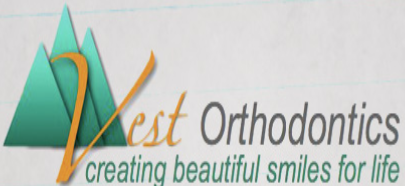The image features a vibrant and eye-catching advertisement for Vest Orthodontics. Set against an off-white or gray background, the banner prominently displays the brand name "Vest" in a stylish yellow-orange cursive font. To the left of the text are three green triangles, representing pine trees, adding a natural and inviting element to the design. Adjacent to "Vest," the word "Orthodontics" is written in a regular black font, maintaining a professional tone. Beneath this, the tagline "creating beautiful smiles for life" is displayed in green, non-script, lowercase letters, likely Helvetica. The overall layout positions the trees on the top left, with the textual elements extending towards the bottom right, making the logo and slogan the focal points. The design utilizes a harmonious color palette of off-white, green, yellow-orange, gray, and black, making it visually appealing and suitable for a company letterhead or business card.